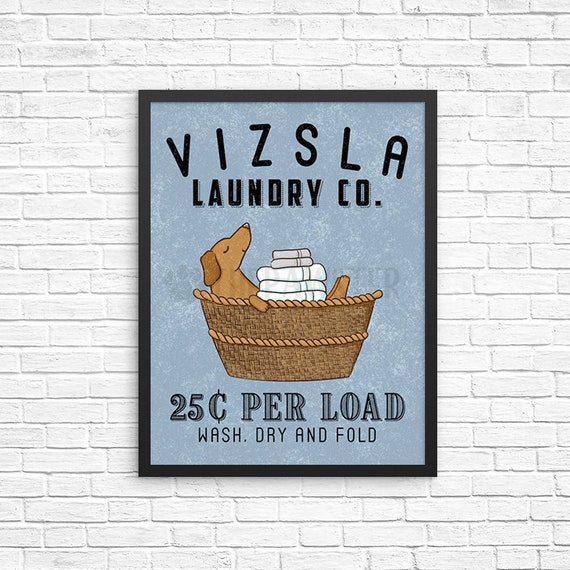The image depicts a framed graphic art poster affixed to a white-painted brick wall with a light gray mortar. The poster's frame is black, and the background is a slate blue with subtle white splashes. At the top of the poster, in bold black letters, it says "VIZSLA Laundry Co." Below this, additional text reads "25 cents per load, wash, dry, and fold." Central to the poster is an illustration of a cheerful brown dog lounging in a tan basket, its nose pointed upward and eyes closed in contentment. The dog has one paw draped over the basket's edge and is covered with folded white towels and embroidered gray rags stacked on its stomach. The intricate details of the dog and the neatly arranged laundry add a whimsical charm to the artwork.